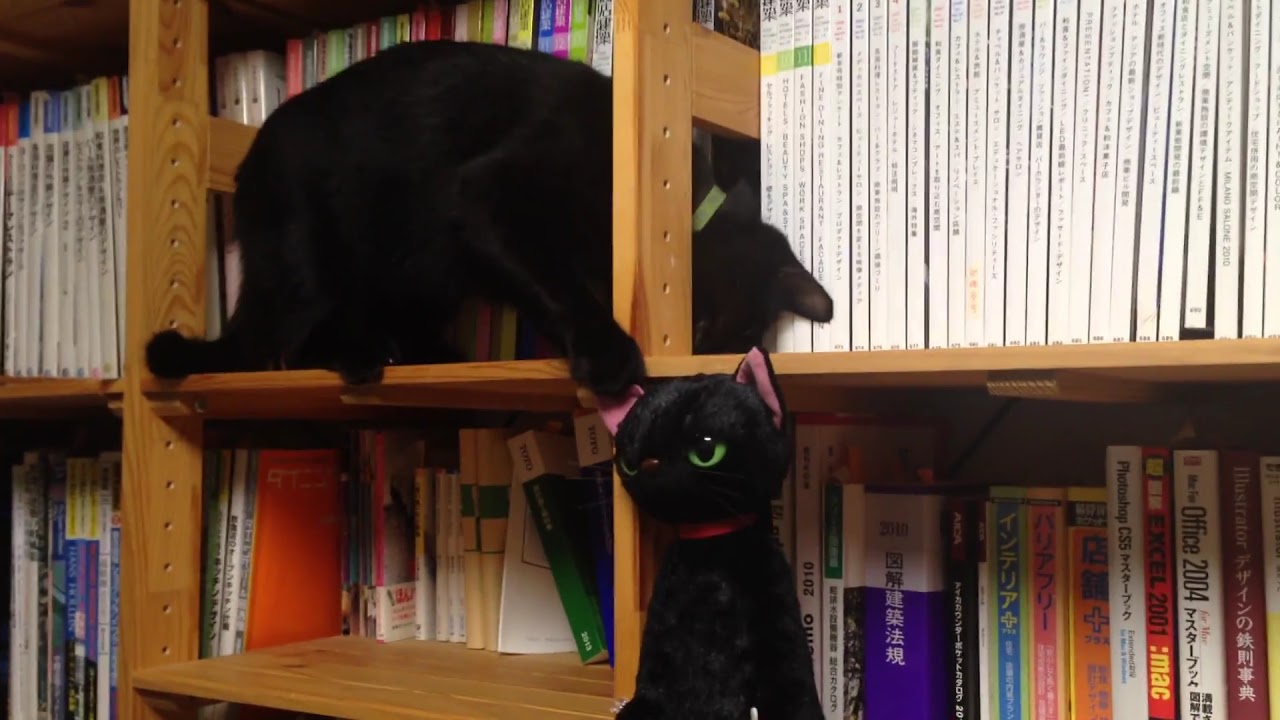This image features a detailed and intriguing scene centered on a black cat and its surroundings. The cat, adorned with a green collar, is positioned on a brown wooden bookshelf that is filled with a variety of books. The assortment includes books in different colors – red, green, pink, purple, white, among others – and features both thick and thin volumes, some with Japanese text on the spines. The cat is interacting with a stuffed animal black cat, identifiable by its green eyes and pink ears, which is positioned on the same shelf. The real cat appears to be pawing at the stuffed animal's pink ear, with its head partially nestled through a gap in the bookshelf’s frame, and its other paw resting near the stuffed animal. The bookshelf itself is designed with small holes drilled throughout its supports, adding a unique touch to the overall structure. This close-up captures a moment of curiosity and interaction between the lifelike cat and its toy counterpart, set against the diverse and colorful backdrop of the books.